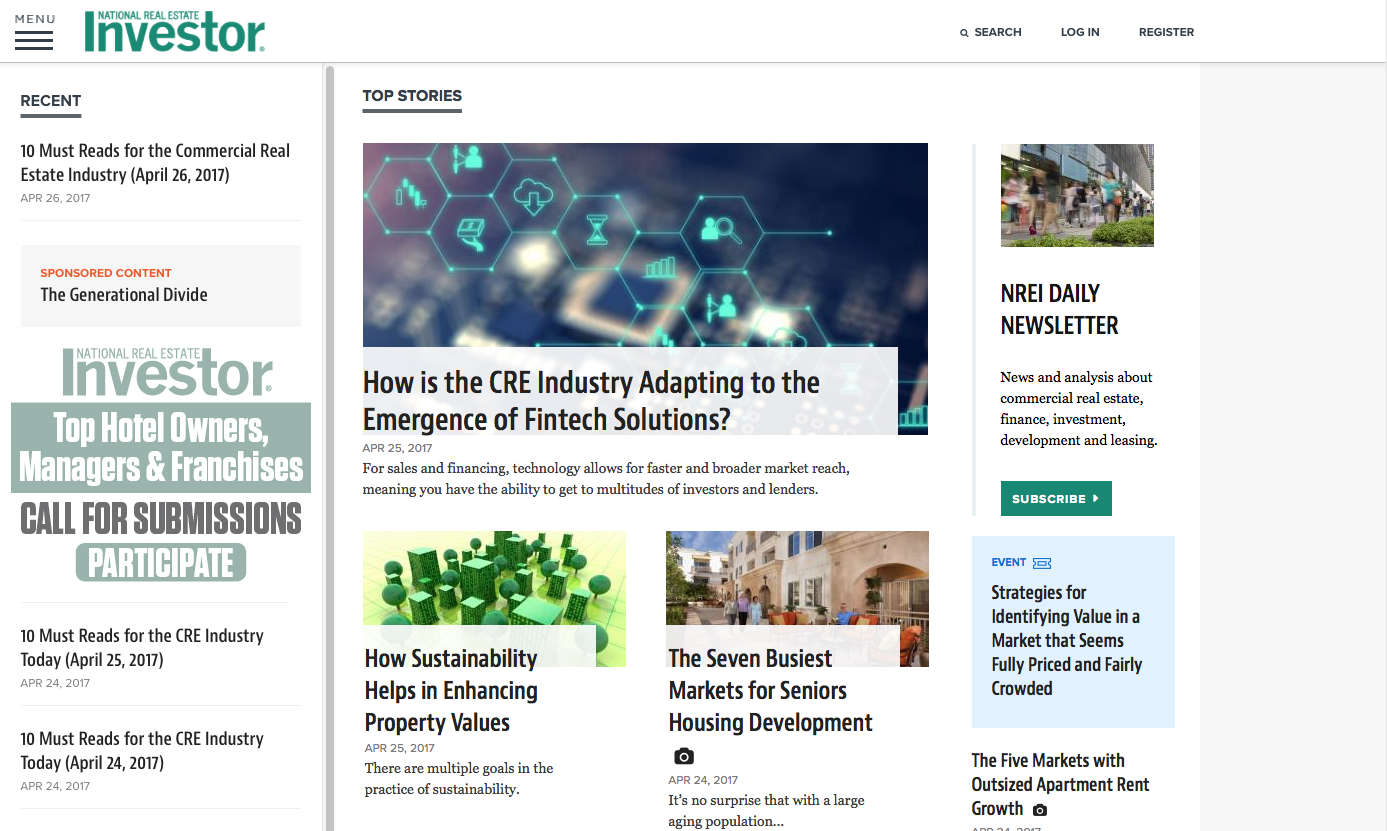This image is a screenshot of an article from the online publication **National Real Estate Investor**. The layout of the website features a clear and organized structure, divided into two main sections: "Recent" and "Top Stories." At the top left, the site displays its logo, company name, and a hamburger menu icon for navigation. On the right, there are options to search the site or log in/register.

The "Recent" section on the left side of the page lists headline news from around April 2017. The "Top Stories" section, which spans from the center to the right, highlights major articles. Notable headlines in this section include: "How is the CRE Industry Adapting to the Emergence of Fintech Solutions?", "How Sustainability Helps in Enhancing Property Values," and "The Seven Busiest Markets for Seniors Housing Development."

The website’s design emphasizes easy navigation and quick access to the latest news and top stories in the commercial real estate industry.